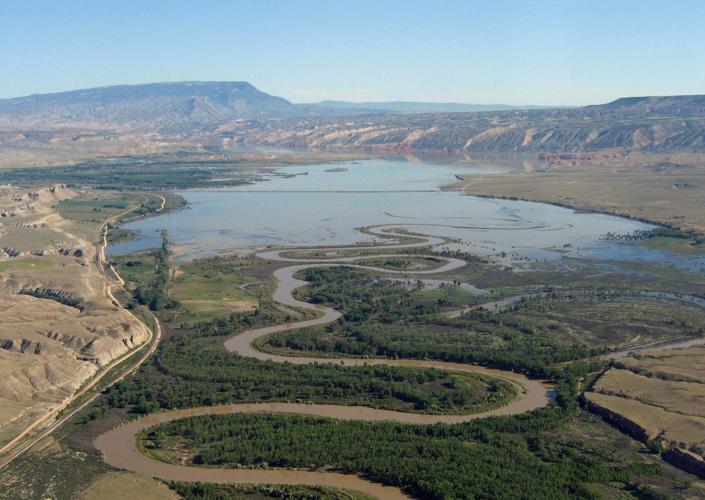This color landscape photo captures a vast, flooded valley under a clear, cloudless blue sky. Low-lying, worn-down brown mountains stretch across the horizon, framing the scene. Dominating the center of the image is a murky brown river, snaking its way from the foreground through lush green trees and dense forest areas. The river meanders in a winding, swirling pattern towards the horizon, eventually merging with a broader body of water that has a subtle blue tint and has inundated the entire valley. In the foreground, green, lush trees thrive between the river bends, but as the valley stretches into the distance, these trees become submerged by the floodwaters. To the right of the image, a grass-covered land juts into the scene, while to the left, taller flat rocks with patches of green moss create a natural boundary. The scene is devoid of any residential structures, emphasizing the untouched, natural beauty of this flooded valley landscape.